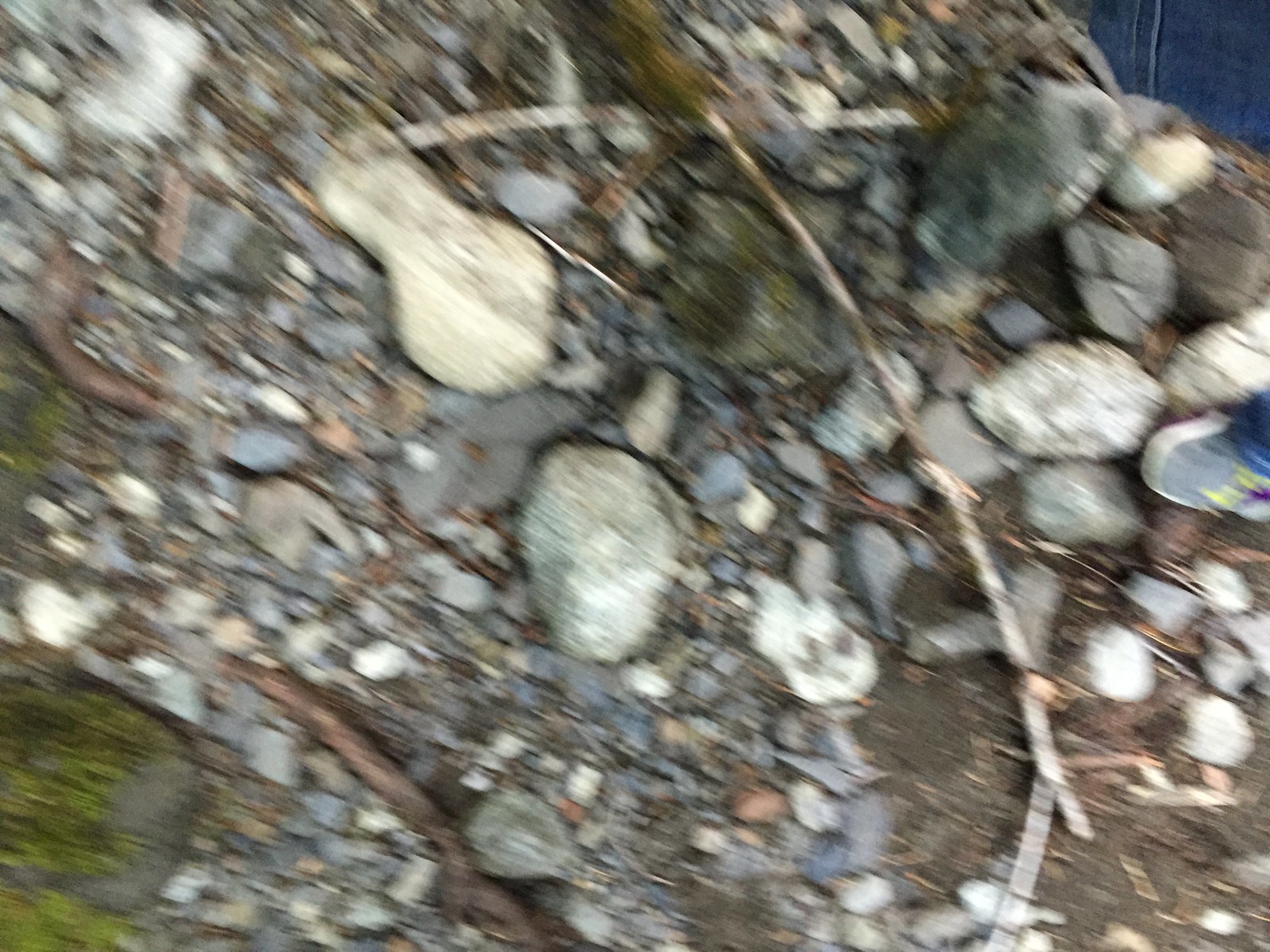This image, though out of focus and likely taken by accident, captures a close-up view of the ground. The terrain is composed of various types of rocks: larger, white stones, smaller pewter-colored pebbles, and a few scattered red rocks. Among the loose earth and stones, a single stick is visible. In the upper part of the frame, a child's foot enters the shot, clad in a small, gray shoe with white accents and yellow laces. Part of the child's denim pant leg can also be seen, adding a contrasting texture and color to the earthy scene.